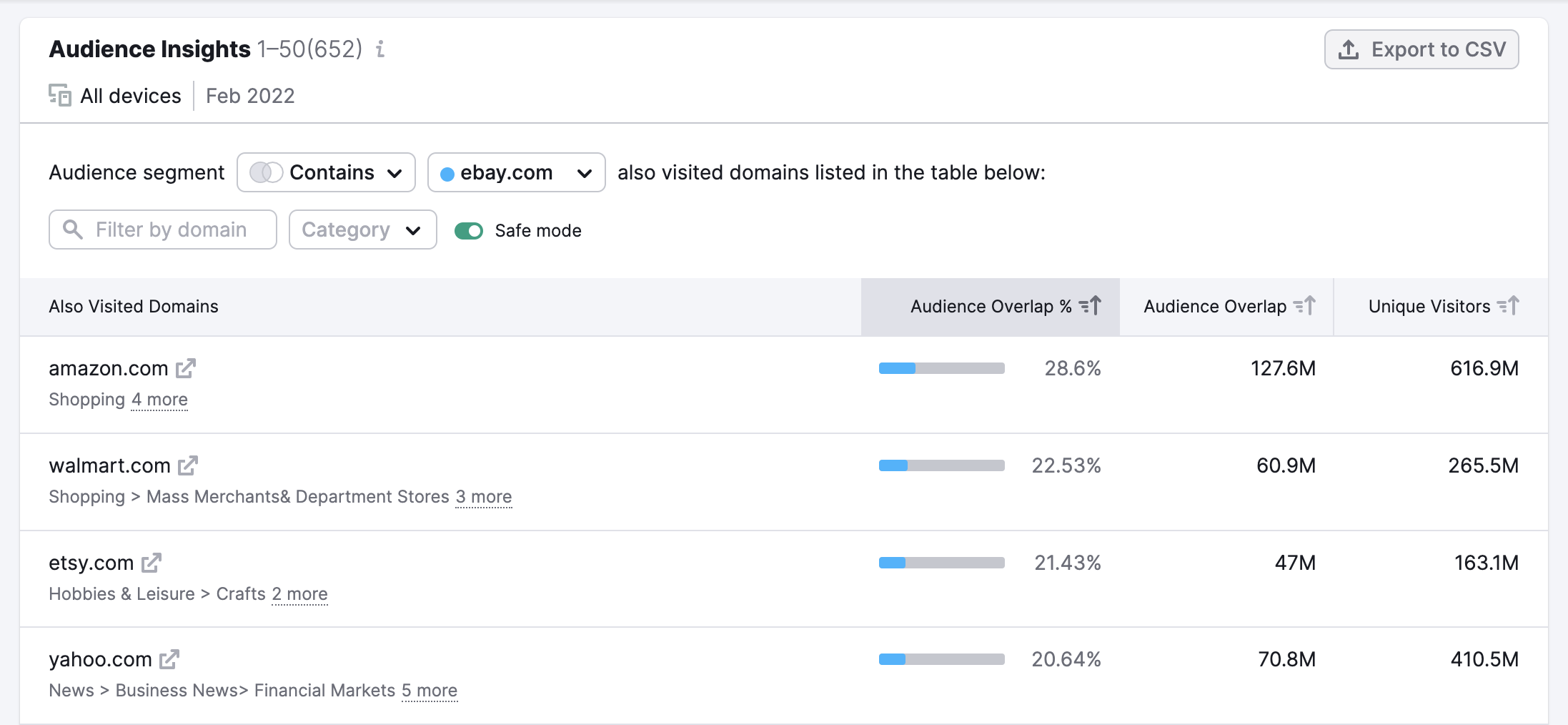**Descriptive Caption:**

The image illustrates a detailed interface of an SEO software focused on providing insights for various websites. 

The interface is contained within a gray box, housing numerous elements. The top section prominently displays "Audience Insights" in bold, dark black font. Next to it appears "1 to 50" with "652" in parentheses, accompanied by an eye icon. On the extreme right, a button labeled "Export to CSV" features an icon of a tray with an up-arrow, indicating the functionality to export data into a CSV format compatible with applications like Excel for organized column and row arrangement.

Underneath this, a line separates the header from the main content. The section below is titled "All Devices," depicted with icons of a computer and a phone, beside "February 2022." A subtle line further segments this area.

The main body starts with a header marked "Audience Segment." Following are segments labeled "Contains" that appear to be part of a join operation in a dropdown format, hinting at options for outer and inner loops. Adjacent is a blue dot labeled "eBay.com," implying a selectable site with a dropdown for choosing other sites. This section emphasizes "Also Visited Domains" and includes a domain filtering option with a category dropdown. Additionally, it shows a "Safe Mode" indicator, switched on and displayed as a green bar.

The table below details "Also Visited Domains" with each website name followed by an icon of a square with an arrow pointing to the upper right corner, indicating an external link. For each domain, data is as follows:

- **Amazon.com**: Shopping
  - Audience Overlap: 28.6%
  - Audience Overlap Count: 127.6 million
  - Unique Visitors: 616.9 million

- **Walmart.com**: Shopping, Mass Merchants, and Department Stores
  - Audience Overlap: 22.53%
  - Audience Overlap Count: 60.9 million
  - Unique Visitors: 265.5 million

- **Etsy.com**: Hobbies and Leisure, Crafts
  - Audience Overlap: 21.43%
  - Audience Overlap Count: 47 million
  - Unique Visitors: 163.1 million

- **Yahoo.com**: News, Business News, Financial Markets
  - Audience Overlap: 20.64%
  - Audience Overlap Count: 70.8 million
  - Unique Visitors: 410.5 million

Each entry includes the audience overlap percentage, the numerical overlap, and the unique visitor count, offering a comprehensive insight into the audience segmentation and overlap across different websites.